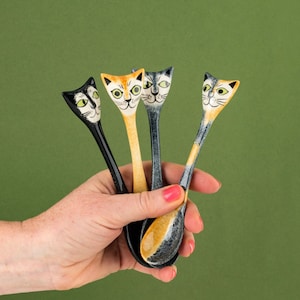In this close-up photograph set against an olive-green background, a hand with peach-colored nail polish is holding four ceramic spoons, resembling a bouquet of flowers. Each spoon has a small eating area, about the size of a thumbprint, and terminates in a uniquely expressive kitty cat head. There is a black cat with a white face, yellow eyes, and black pupils; an orangish-yellowish cat with a similar white face and yellow eyes with black pupils; a gray cat with a white face and green eyes; and a calico cat with a white face and green eyes. The facial expressions of these cat heads vary, with some looking to the left and some looking forward. The spoons are painted to match the cats at their ends, with two spoons being predominantly dark black, and the other two being shades of orangish-beige mixed with black. The hand holding these spoons has relatively short nails, further emphasizing the intricate details of the charming cat spoon set.